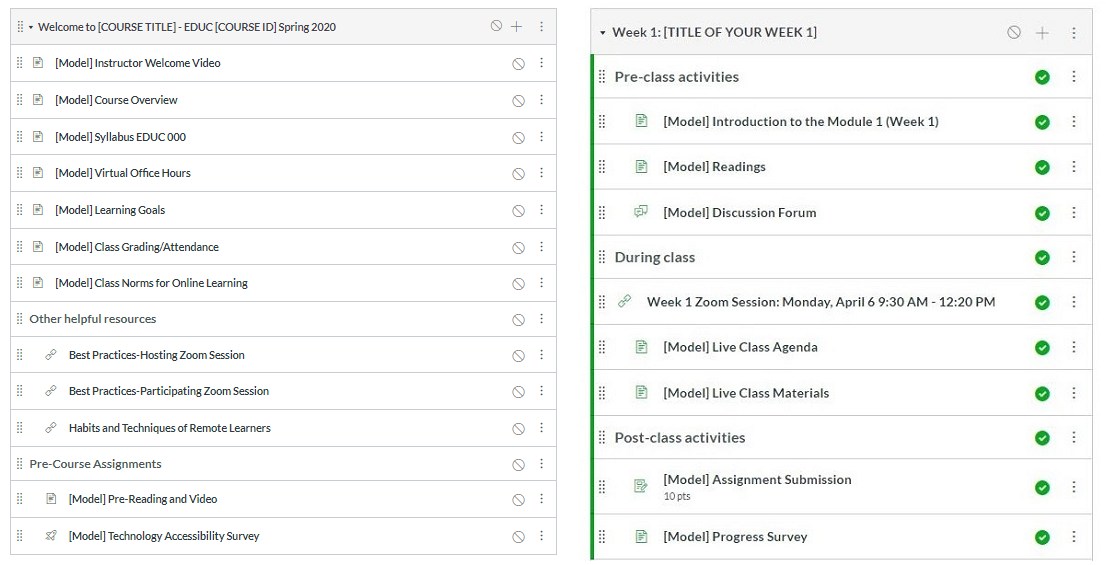**Descriptive Caption:**

The interface is divided into two columns, each serving a specific organizational purpose. 

**Left Column:**
- **Title and Course Information:** "Welcome to Course Title - EDUC, Course ID Spring 2020."
- **Modules:** These are sequentially listed from top to bottom:
  1. Instructor Welcome Video
  2. Course Overview
  3. Syllabus (EDUC 000)
  4. Virtual Office Hours
  5. Learning Goals
  6. Class Attendance
  7. Classroom for Online Learning
- **Other Helpful Resources:** 
  - Best Practices for Hosting Zoom Sessions
  - Best Practices for Participating in Zoom Sessions
  - Syllabus and Techniques for Remote Learners
- **Pre-course Assignments:** 
  - Pre-learning Video
  - Technology Accessibility Survey

**Right Column:**
- **Week One:** The heading indicates the start of the first week.
  - **Pre-class Activities:** All items listed here have green check marks, indicating completion. 
    1. Instructor Module for Week One
    2. Assigned Readings
    3. Discussion Forum
  - **During Class:** 
    - Week One Zoom Session scheduled for Monday, April 6th, from 5:30 AM to 12:20 PM
    - Live Class Agenda
    - Live Class Materials
  - **Post-class Activities:**
    - Assignment Submission
    - Progress Survey